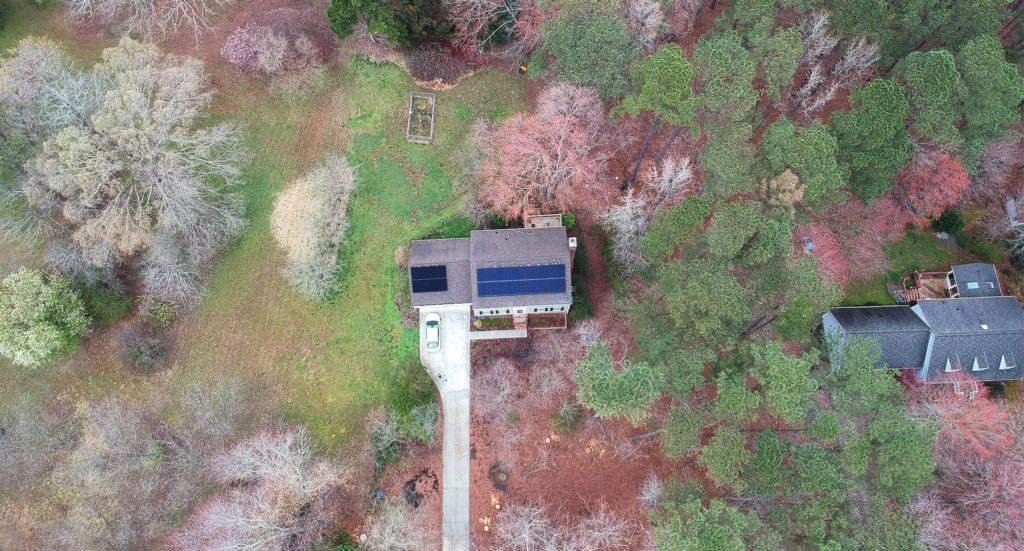This is a professionally taken aerial photograph showcasing a piece of property in a landscape view. Central to the image is a main house with a gray roof that features blue solar panels. Extending from the house is a long whitish light gray driveway, where a white car is parked. To the right is a second house with a dark gray roof and an additional extension that features a canopy at the front and windows visible on the upper level.

Surrounding the houses are vibrant fall trees in an array of colors, including shades of green, pink, red, burgundy, and white. The ground on the right side of the image is notably covered in pinkish-red dirt, contrasting with the fading green grass and patches of pink grass in the upper left corner. Additionally, there is a small square that appears to be a garden in the backyard, and a stack of white objects in the yard. The verdant and diverse foliage, some of which resembles broccoli from this angle, and the general landscape indicate a picturesque setting that might be captured for a real estate listing.